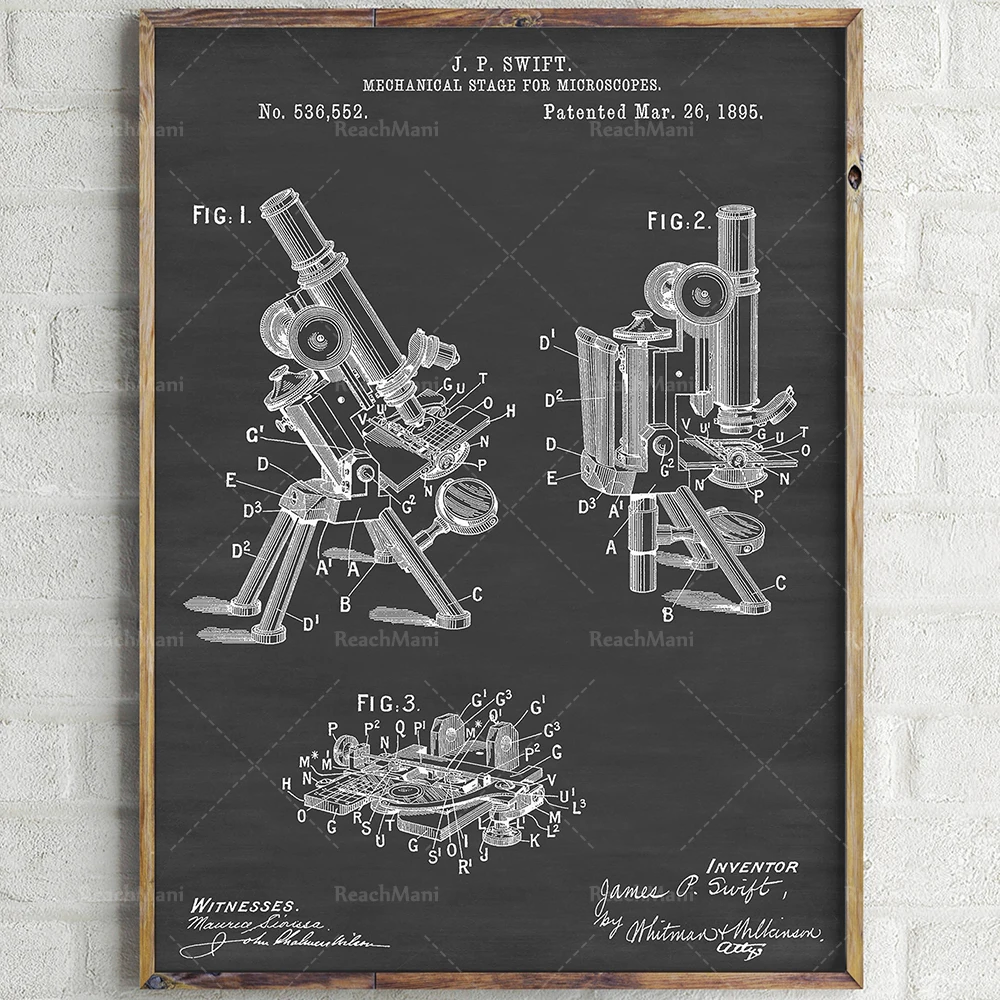The image is a detailed sketch diagram of various microscopes, mounted within a wooden frame against a brick wall, either light gray or white. The diagram itself has a black background with white text and illustrations. At the top, it prominently features the title "J.P. Swift Mechanical Stage for Microscopes," along with patent number "536552" and the date "Patented March 26, 1895." The diagram includes three figures of microscopes, each accompanied by labels pointing to different parts. Figure 1 and Figure 2 are depicted on the left and right, respectively, while Figure 3 sits centrally below them. Towards the bottom left corner, the diagram lists names under the heading "Witnesses," whereas the bottom right corner is signed with "Inventor James P. Swift by Whitman." Additional text, possibly including the words "REACH MANNY," is present but partially obscured or unclear.